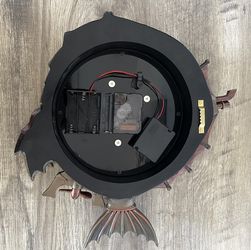The image displays the exposed interior of a black power saw, viewed from above within a small square frame. The circular device, with its cover removed, reveals intricate electronic components. At the center, two rectangular batteries are connected by red wires, extending to a third gray battery. Adding to the complexity are three round holes, placed at the upper middle, slightly lower to the right, and at the bottom middle of the device. The prominent serrated blade can be seen in the lower left section of the saw, with additional smaller blades positioned towards the top. A peculiar, almost fishtail-like extension protrudes from beneath the saw. The device rests on a light gray wooden surface, suggesting it may be undergoing maintenance or repair. Gold writing is visible along the right edge of the black casing, and the overall scene combines a technical focus with a backdrop of tactile wood.